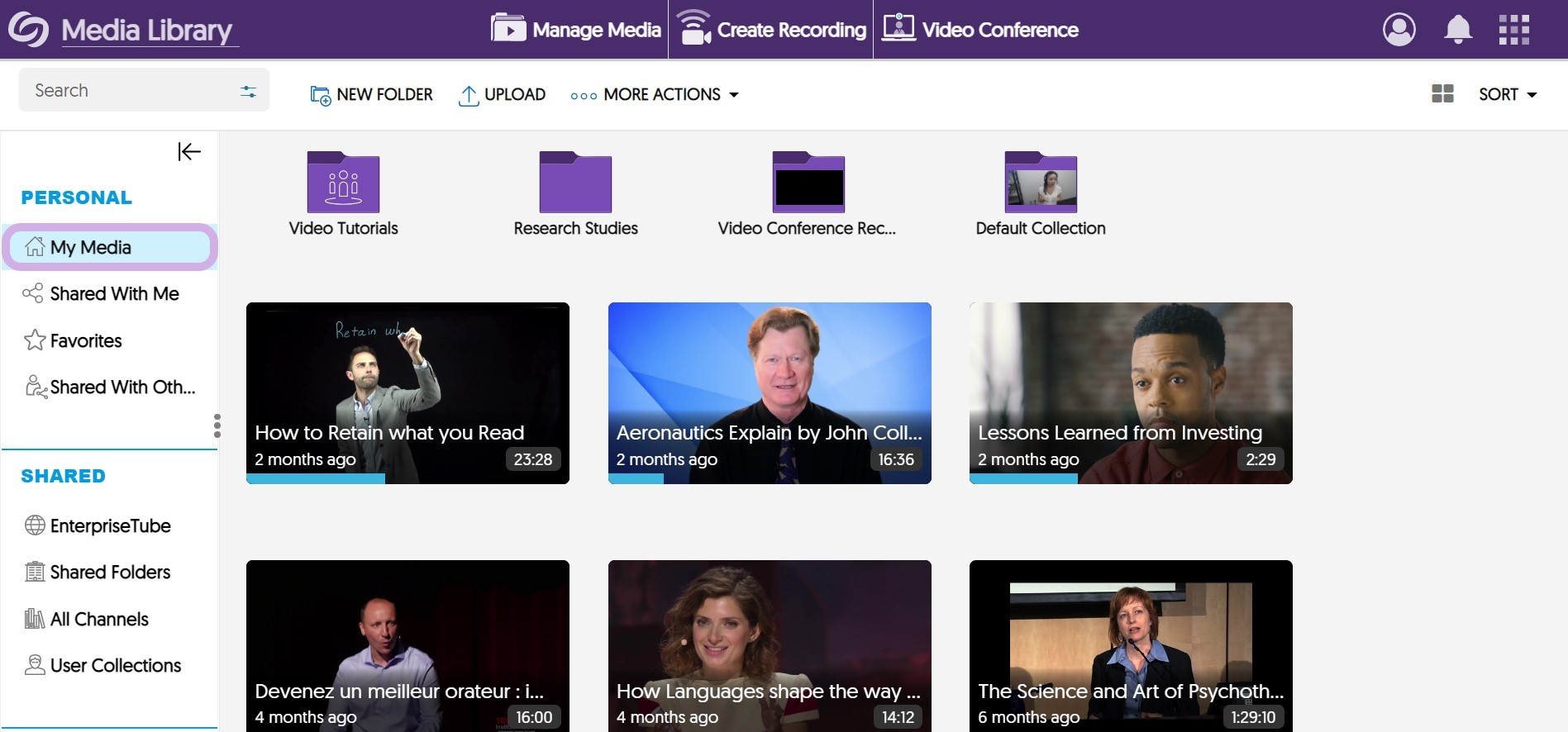This detailed rectangular horizontal screenshot captures a Media Library interface on a cell phone. Predominantly featuring a purple theme, the top part of the screen displays the application’s logo alongside the bold text "Media Library". Prominently centered below the header is an icon symbolizing media management labeled "Manage Media," accompanied by a video icon with Wi-Fi bars above it that says "Create Recording". Adjacent to it, a laptop icon signifies the "Video Conference" feature.

In the top right corner, the user interface presents a user symbol, a bell icon for notifications, and a clickable grid menu. Just below "Media Library" on the left, there's a search bar for finding media within the library. Following it, clickable options for "New Folder," "Upload," and "More Actions" are neatly lined up. On the right, beneath the purple bar, there is a grid view toggle labeled "For Grid" and a sortable dropdown menu for organizing content.

The left sidebar of the page comprises two sections: "Personal" and "Shared." Under "Personal," options like "My Media," "Shared with Me," "Favorites," and "Shared with Others" are listed, with "My Media" currently selected. The "Shared" section further segregates content into "EnterpriseTube," "Shared Folders," "All Channels," and "User Collections."

The main content area showcases four purple folders labeled "Video Tutorials," "Research Studies," "Video Conference Recordings," and "Default Collection." Six videos are displayed below these folders:
1. "How to Retain What You Read" - posted two months ago.
2. "Aeronautics Explained by John" - posted two months ago.
3. "Lessons Learned from Investing" - posted two months ago.
4. A 60-minute video in another language - posted four months ago.
5. "How Languages Shape the Way" - posted four months ago.
6. "Science and Art of Psychotherapy" - posted six months ago.

This screenshot offers a comprehensive glimpse into the organized features and extensive media content available in the Media Library application.